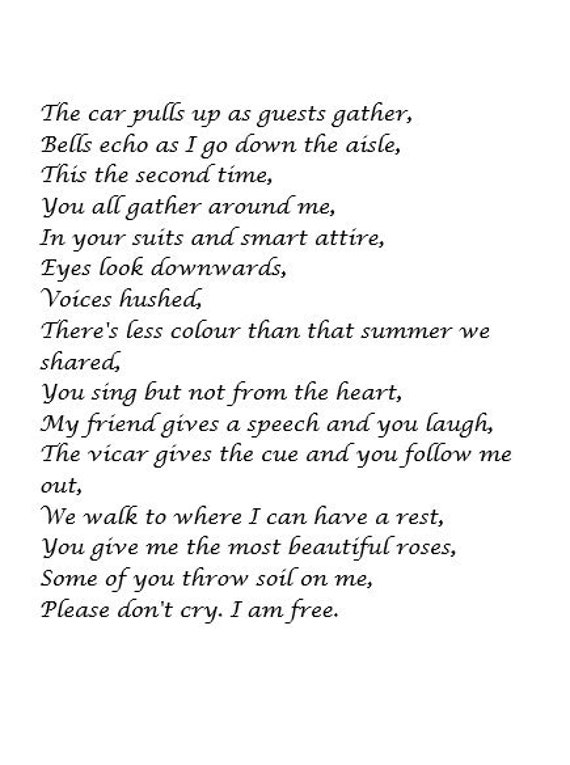The image captures the poignant verses of a poem penned in an elegant, flowing script. Initially, the poem mirrors the ambiance of a wedding, with mentions of guests arriving at a church and the author describing the walk down the aisle. However, as the poem transitions, it becomes evident the subject is not a wedding but a somber funeral. The author corrects the initial impression, indicating the ceremony is in fact a farewell, with lines like "some of you throw soil on me" and a heartfelt plea, "Please don't cry. I am free." The vulnerability and depth of emotion in the poem's revelations evoke a deep sense of melancholy and liberation, capturing the complex feelings surrounding a final goodbye.